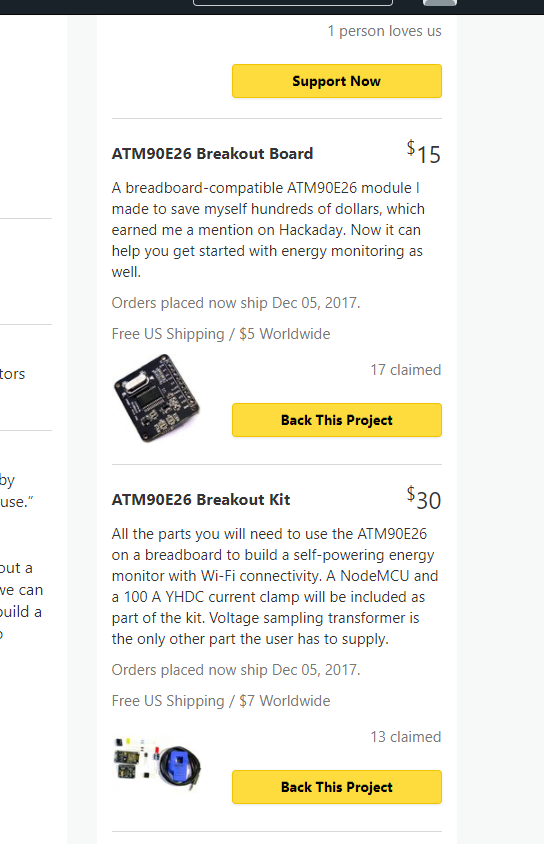This image showcases a cropped section of a crowdfunding website, resembling platforms like Indiegogo, where inventors present their products for pre-order. The website features a grey background, divided into sections for different product listings.

On the left side of the image, there is the right edge of a large white box. Adjacent to this is a wide space followed by a vertical rectangular white box to its right. At the top left of this box, the text "One Person Loves Us" is displayed in small grey font. Below this, a bright yellow rectangular button with bold black text reads "Support Now."

Below this section is a thin grey horizontal line. Beneath the line, a product listing begins with the title "ATM90E26 Breakout Board" in bold black font on the left, priced at $15 on the right. This is followed by a brief description of the product. Below the description, the text indicates that orders placed now will be shipped on December 5th, 2017, with free shipping in the US and a $5 worldwide shipping fee. At the bottom left of this listing, there is a small image of the product. To the right of the image, the text "17 claimed" appears in small grey font. Below this, another rectangular yellow button with black text reads "Back This Project."

Further down, there is another product listing for an "ATM90E26 Breakout Kit" priced at $30. This listing also includes a brief product description. At the bottom left, small images of the product are displayed, and to the right of these images, "13 claimed" is noted. At the bottom right, there is another rectangular button that says "Back This Product."